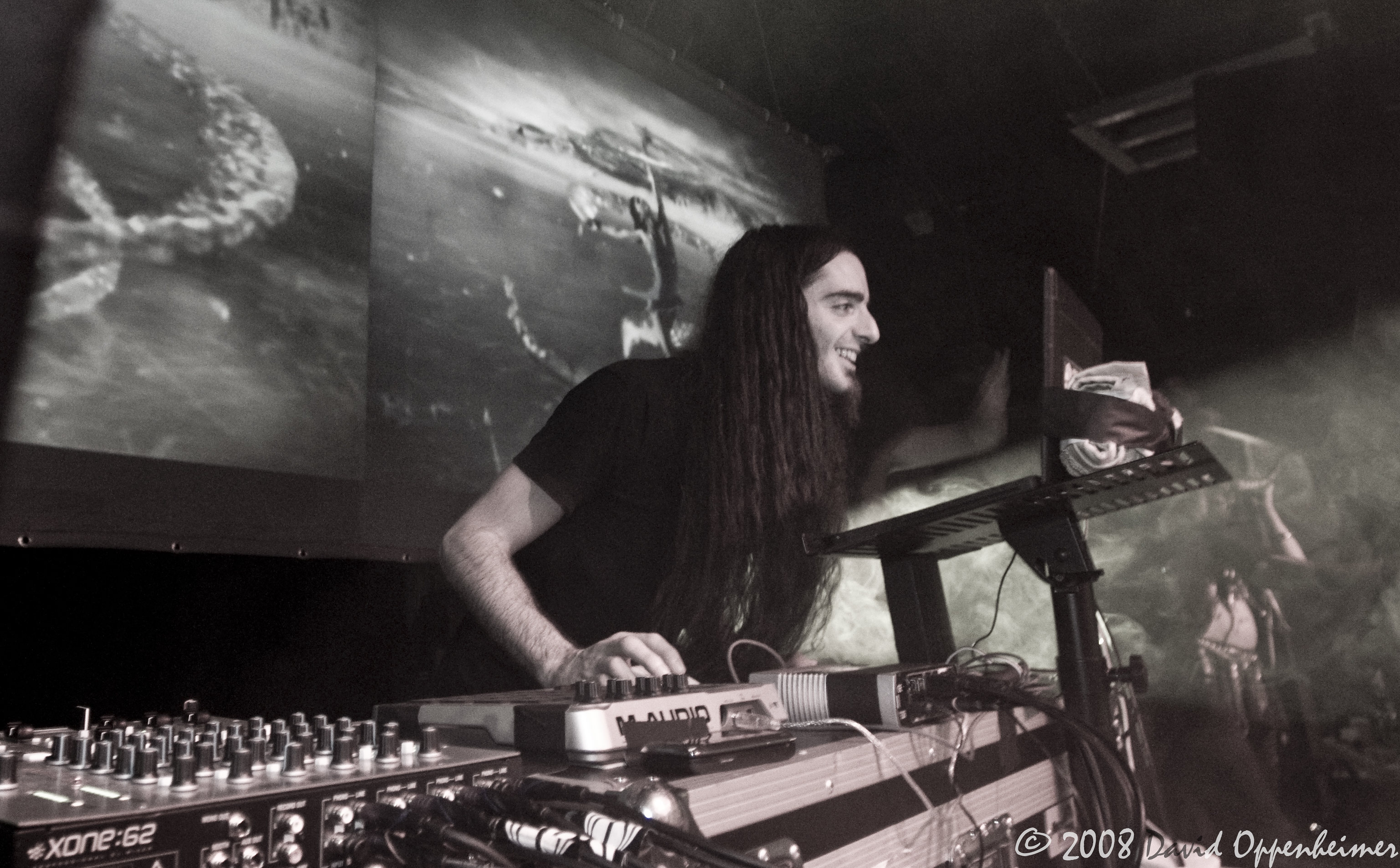This striking black and white photo captures a man with very long dark hair, a large nose, and a smiling face, as he stands in the midst of a concert, facing to the right. He is wearing a short-sleeved black t-shirt and operates a soundboard filled with numerous black knobs, with a metal stand holding a laptop in front of him. A gigantic screen behind him displays projected images, including what appears to be water or an ocean on the left, and a dancing woman on the right. The scene is indoor and suffused with a smoky or foggy atmosphere, possibly from a fog machine. Positioned nearby, another band member stands near a microphone, with a crowd of people visible behind him. The lower left-hand corner of the photo displays the label "XONE-62" on the control panel, while the bottom right-hand corner bears the copyright mark, "2008 David Oppenheimer."